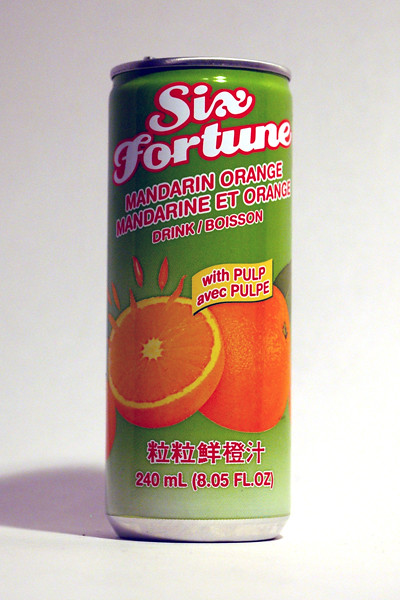The image showcases a drink product placed on a pristine white surface. The scene is illuminated in a way that casts a distinctive shadow of the drink product. The product itself is a can, predominantly green in color with silver accents at the top and bottom. Prominently displayed on the can in bold white lettering, outlined in red, is the brand name "Six Fortune." Below it, in contrasting red text outlined in white, it reads "Mandarin Orange." Additionally, there is text in another language, followed by the word "drink," and a note stating "With Pulp."

The can is adorned with vibrant graphics, including two Mandarin oranges – one whole and the other cut open, revealing juicy segments with splashes of the tangy fruit visible. Asian characters in white and red are also present, adding a distinctive cultural touch. Towards the bottom of the can, the volume is specified in white text: "240 ml (8.05 fl. oz.)."